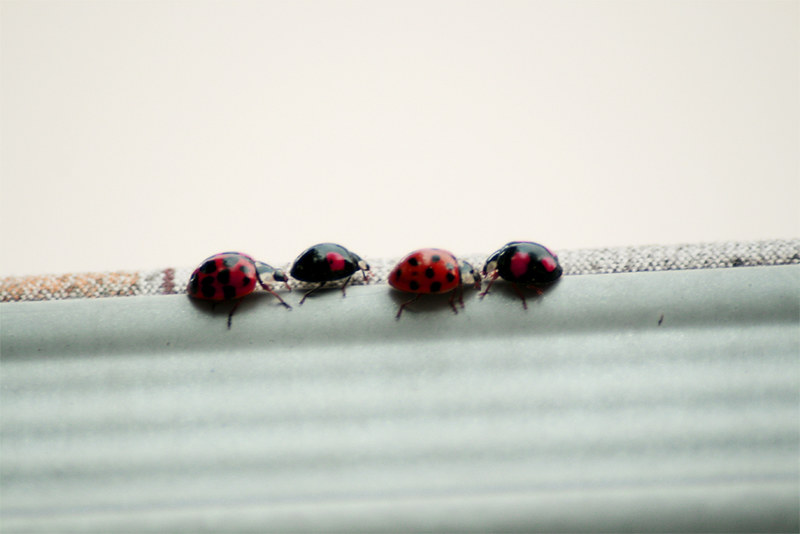This vibrant, landscape-oriented image showcases four beetles of the order Coleoptera, commonly referred to as ladybugs, lined up horizontally along what appears to be the edge of a white surface, possibly outdoor furniture or a piece of clothing, with beige patterned fabric in the background. Each beetle displays distinct coloration: the first and third beetles from the left have striking red shells adorned with black dots, with the first beetle's large, almost-touching dots standing out. The second and fourth beetles, however, feature primarily black shells with red splotches. Observing their orientation, the first beetle faces left while the others face varying directions; the second beetle faces towards the center, the third beetle to the right, and the fourth beetle also towards the center. Their different dimensions and spot patterns hint at potential variations in species or gender.